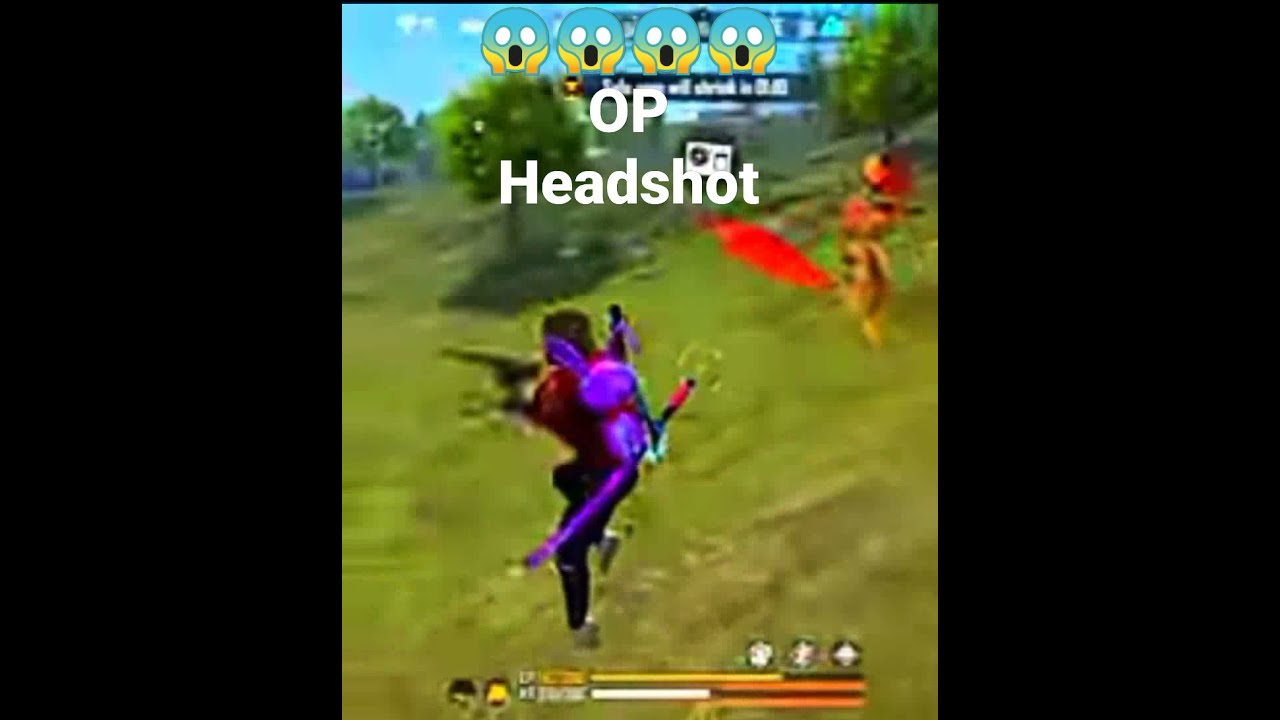This wide rectangular image features a tall rectangular screenshot from a low-resolution video game, framed by black bars on the left and right. Central to the image is a character, slightly left of center, wearing dark, form-fitting pants and a red top, equipped with a neon-lit purple backpack and an attached weapon. The character appears to be running away from the screen on a lush, green, slanted hill. Surrounding the hill are large, leafy green trees that stretch towards a sky painted in bright blue with small white clouds. Slightly above and to the right of the character, an orange and black bug, possibly a bee, flaunts a bright red tail. Dominating the top of the screen, in white font, is the text "OP Headshot." Despite the image's heavy compression and low resolution, which render many details indistinct, the vibrant colors of black, green, yellow, orange, purple, teal, and light blue stand out. Additionally, the scene seems to depict two characters, with the main one in the forefront and another, more difficult to discern figure, possibly with a yellow body and orange head, positioned further back.